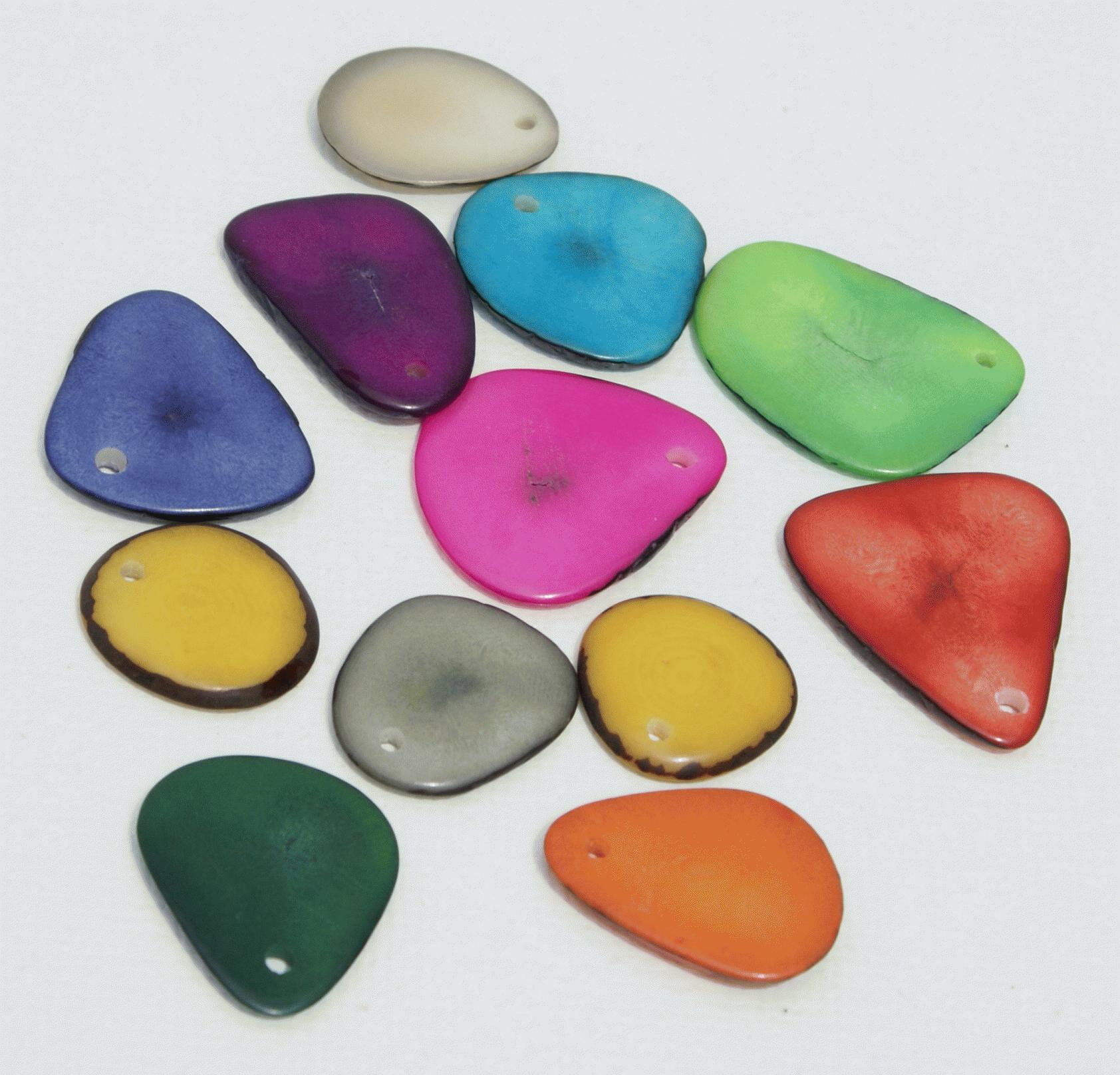A vibrant array of polished, flat stones, shaped like guitar picks and each featuring a small hole for threading into jewelry, is displayed against a pristine white background. The stones, arranged in a somewhat circular pattern, boast a rich spectrum of colors. These include a marble-like off-white stone, deep purple, lavender, turquoise blue, kiwi green, bright pink, solid orange, jade green, and a unique faded red with lighter accents. Additionally, there are two yellow stones with brown edges, and one each of gray and dark blue. Their refined surfaces and variety of hues suggest a meticulous process to prepare these minerals for creating necklaces or bracelets, offering a blend of smooth polish and inherent stone texture that adds to their charm.